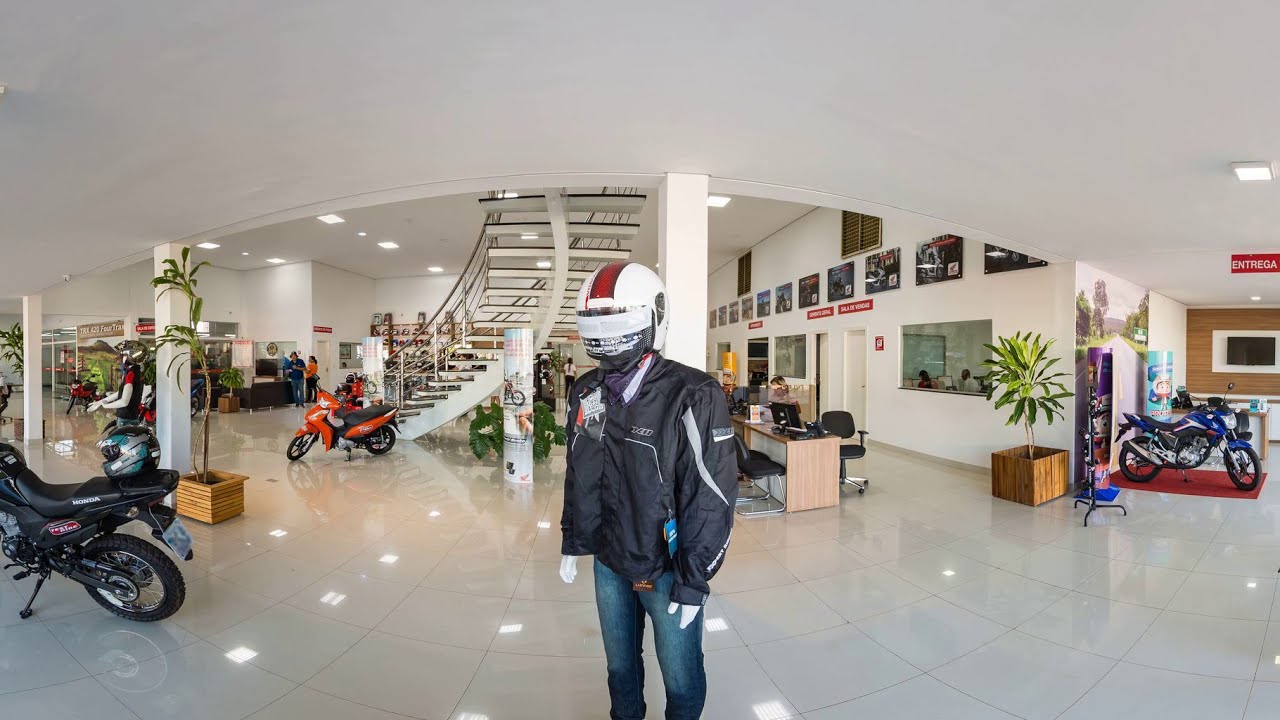In the image, we see a sleek, modern motorcycle showroom dominated by a pristine, white interior. The floor, walls, and ceiling are all brilliantly white, creating an immaculate and almost futuristic environment. The glossy white floor is highly reflective, mirroring the showroom's details and enhancing its luminous quality.

At the center and in the foreground, there's a mannequin dressed in a biker's ensemble, featuring a black motorcycle jacket, blue jeans, and a striking white helmet adorned with a red stripe flanked by thin blue stripes on either side. This mannequin stands as a focal point amidst a variety of motorcycles.

To the left, there is a black motorcycle with a helmet resting on its backseat. Next to this bike, a plant in a box adds a touch of natural greenery, and behind it, another mannequin is visible, similarly geared up for riding. Beyond the planter, an orange motorcycle is positioned close to a spiral staircase that elegantly ascends to an upper level. The staircase features a center section with steps splitting off in an artistic design.

On the right side, another blue motorcycle is showcased. Near this bike, a desk with chairs suggests an area for customer interactions or consultations with a dealer. Moving further right, the image shows a wall with office spaces behind it, adding depth to the showroom's layout. Another plant in a box is situated near the edge of the image, complemented by yet another motorcycle.

The ceiling above, possibly the floor of an upper level, is low and curved, contributing to the showroom's contemporary architecture. Along the top walls, various images are displayed, adding visual interest and branding elements to the space. This meticulously arranged showroom, free of people except for the mannequins, emphasizes the presentation of the motorcycles and the stylish equipment associated with them.